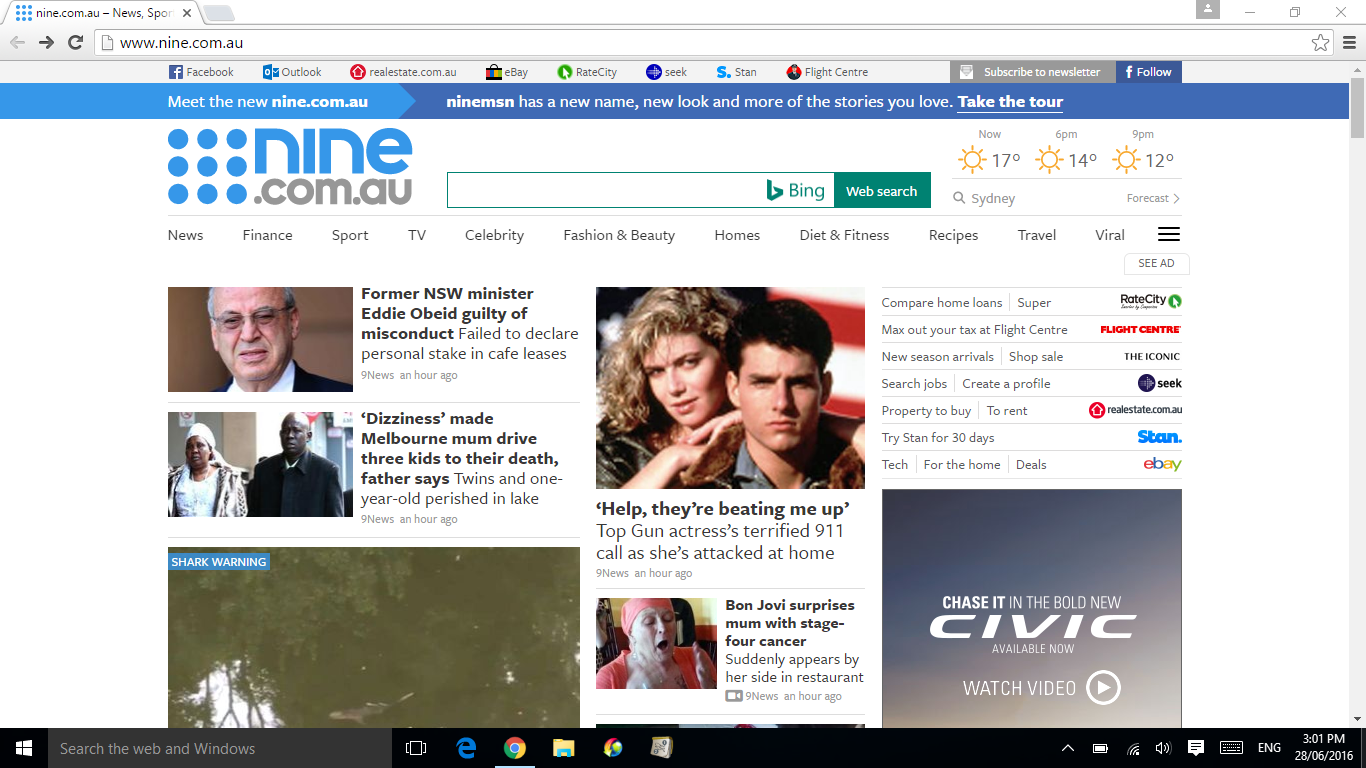This is an image showcasing a revamped homepage of 9.com.au, highlighted by a conspicuous search bar at the top. Upon closer inspection, multiple open tabs are visible, including Facebook, Outlook, RealEstate.com, eBay, Rate City, Seek, Stan, and Flight Center. Below the search bar, a prominent banner introduces the new 9.com.au, rebranded from 9 MSN, emphasizing a fresh design and enhanced content with the slogan "Meet the new 9.com.au: 9 MSN has a new name, a new look, and more of the stories you love. Take the tour."

The website categories stretch out comprehensively, covering widely varied topics such as web search, news, finance, sport, TV, celebrity, fashion and beauty, homes, diet and fitness, recipes, travel, and viral content. An additional expandable menu bar is also present for more navigation options.

The main highlighted story features a report on former NSW minister Eddie Obeid being found guilty of misconduct. Other stories are also prominently displayed, including a tragic account of a Melbourne mother whose dizziness led her to drive her three children to their deaths, an appeal from a father, “Help, they’re beating me up,” and a distressing 911 call from a 'Top Gun' actress, who was terrified as she was attacked at her home.